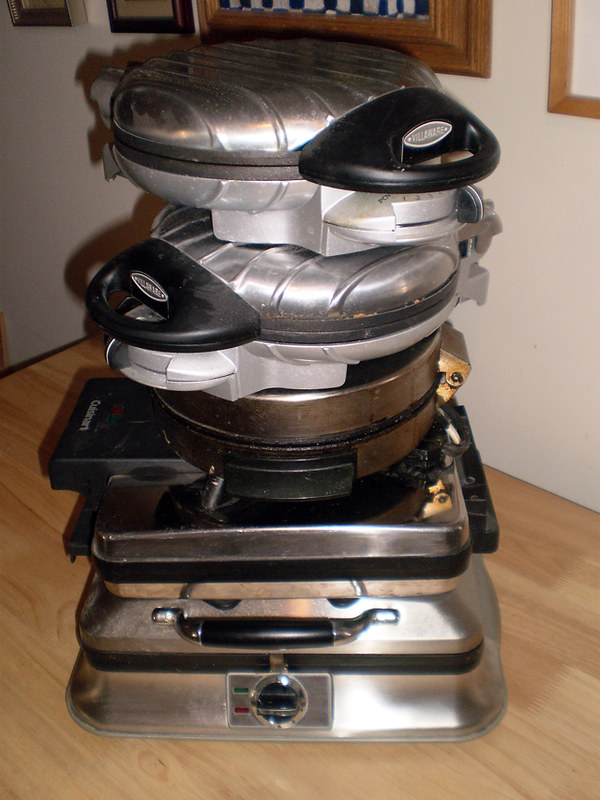The image depicts a stack of five waffle irons on a beige wooden surface. The bottom iron is a chrome square model featuring a metal nozzle, a black handle with metal siding, and dual green and red indicator lights. Positioned above it is a smaller silver rectangular iron with black ends. The third in the stack is a used and slightly rusted Cuisinart Belgian waffle maker, bearing visible signs of grease and grime, also equipped with red and green indicator lights. The fourth and fifth waffle irons are nearly identical circular models with silver lids, black lifting handles, and noticeable usage marks and stains. Both feature a striped pattern. In the background, there is a white wall adorned with several wooden-framed photos, with the shadows of the waffle irons cast on the wall to the left.